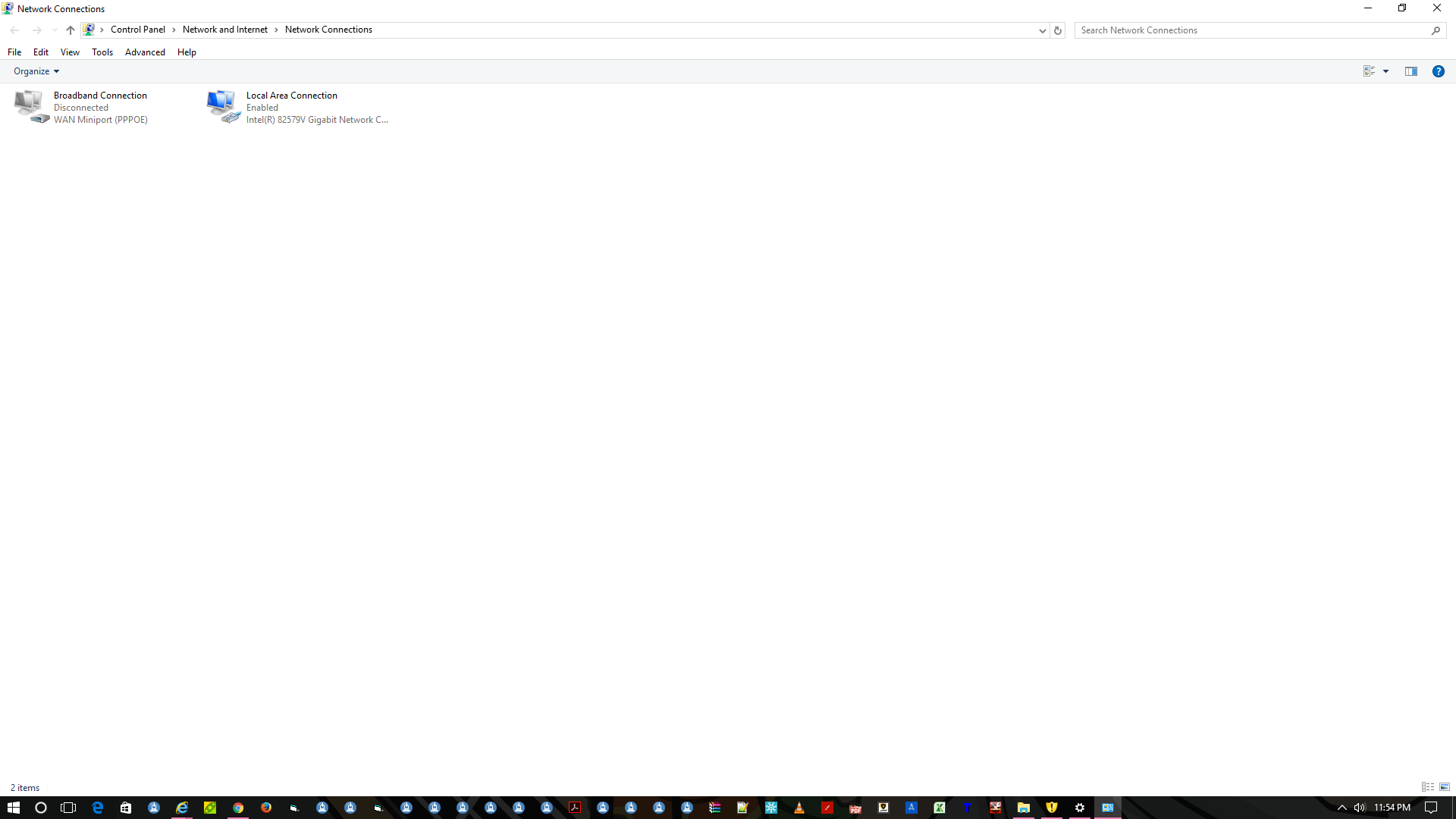The image is a screenshot of a computer desktop. At the top of the screenshot, the title "Network Connections" is visible. The network connections list includes a "Broadband Connection" labeled as disconnected, with an error message referring to "Many poor PPPOE." Below that, there is a "Local Area Connection" which is enabled, specifically identified as "Intel(R) 82579V Gigabit Network."

The screenshot also shows the Windows taskbar at the bottom of the desktop, which is cluttered with an unusually high number of programs—around 30—either open or pinned, making the taskbar look congested and cluttered. The standard Windows interface elements are present, including the search bar at the top, the minimize, maximize, and close buttons (depicted by a right arrow and an 'X') on the top right of the window, and the Windows symbol on the bottom left. Overall, beyond the network connection details, the desktop setup appears standard with the exception of the overfilled taskbar.